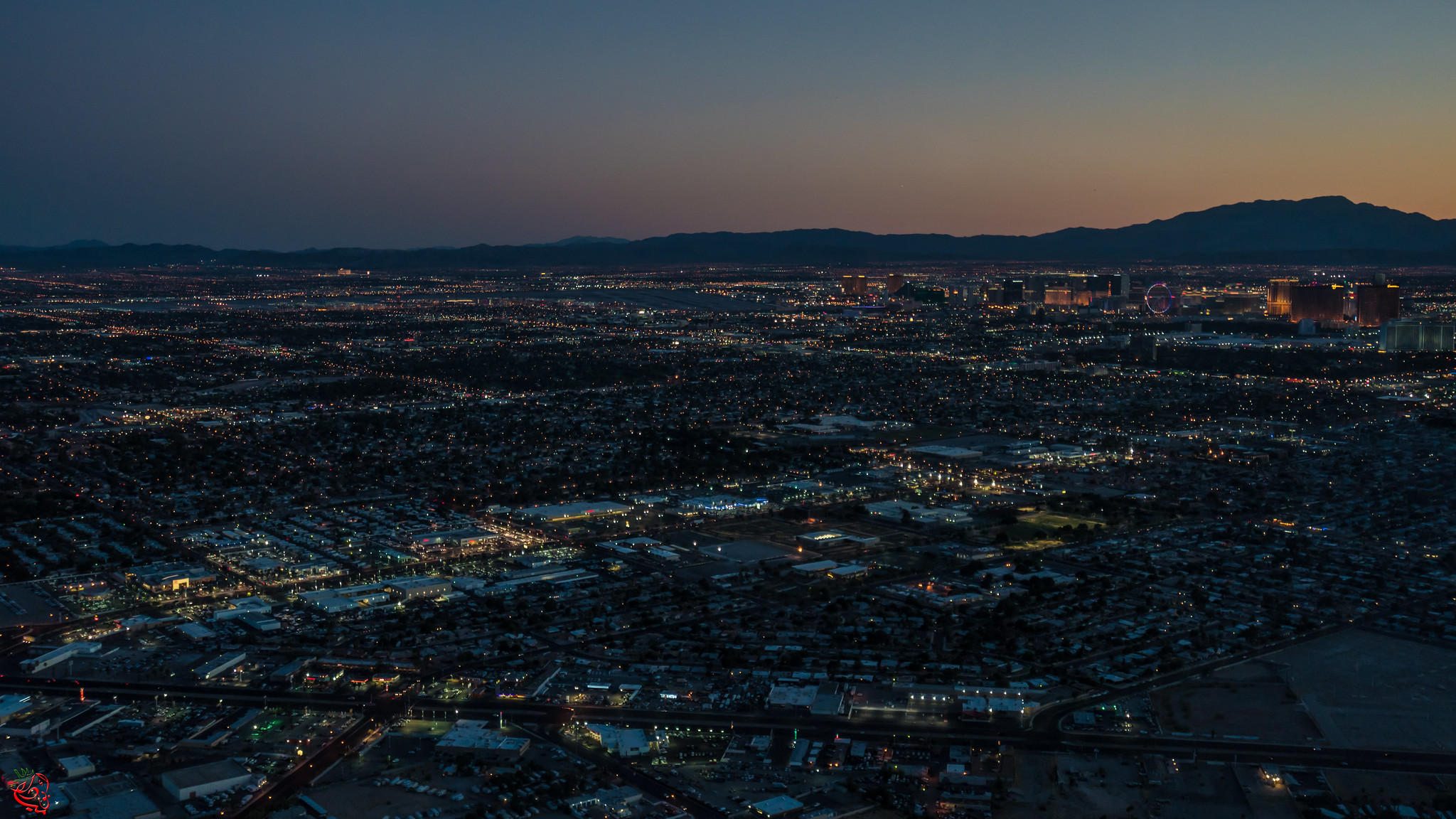This panoramic photograph captures a city nestled in a flat valley, taken just after sunset. The sky is predominantly dark, but a band of vibrant red lingers near the horizon, silhouetting the distant hills, while remnants of blue sky fade into the twilight. The valley is filled with large commercial buildings featuring illuminated windows and extensive flat roofs, particularly prominent in the foreground. In the background, multi-story structures suggestive of hotels or office buildings rise on the right side of the image, contributing to the cityscape's complexity. Central areas interspersed with trees and dotted with small lakes hint at residential neighborhoods, creating a blend of urban and natural elements. Dominating the lower portion of the frame, a four-lane freeway stretches horizontally across the scene, emphasizing the city's infrastructure. Marked by a small strawberry logo in the bottom left corner, the image is tinged with the photographer's unique signature.